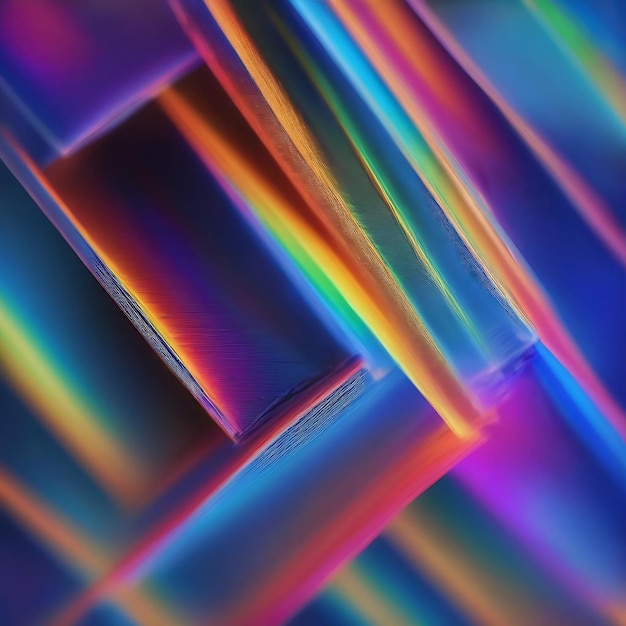A vibrant, highly magnified image showcases an intricate and colorful structure that evokes both natural crystalline formations and abstract digital art. Dominated by striking colors, the scene features a prominent yellow tip that transitions into darker orange hues, giving way to vivid violet and bright orange sections that appear to be backlit for an almost electric effect. Patches of light green and blue accentuate the composition, with a green tubular form turning orange at the image's right edge. The structure itself comprises interconnected, slightly irregular rectangular bars that appear nearly translucent and exhibit neon-like qualities, resembling an array of glowing glow sticks. The overall aesthetic is both dynamic and mesmerizing, with layers of bluish-purple beams bordered by vibrant yellow lines, creating a complex and colorful geometric pattern.